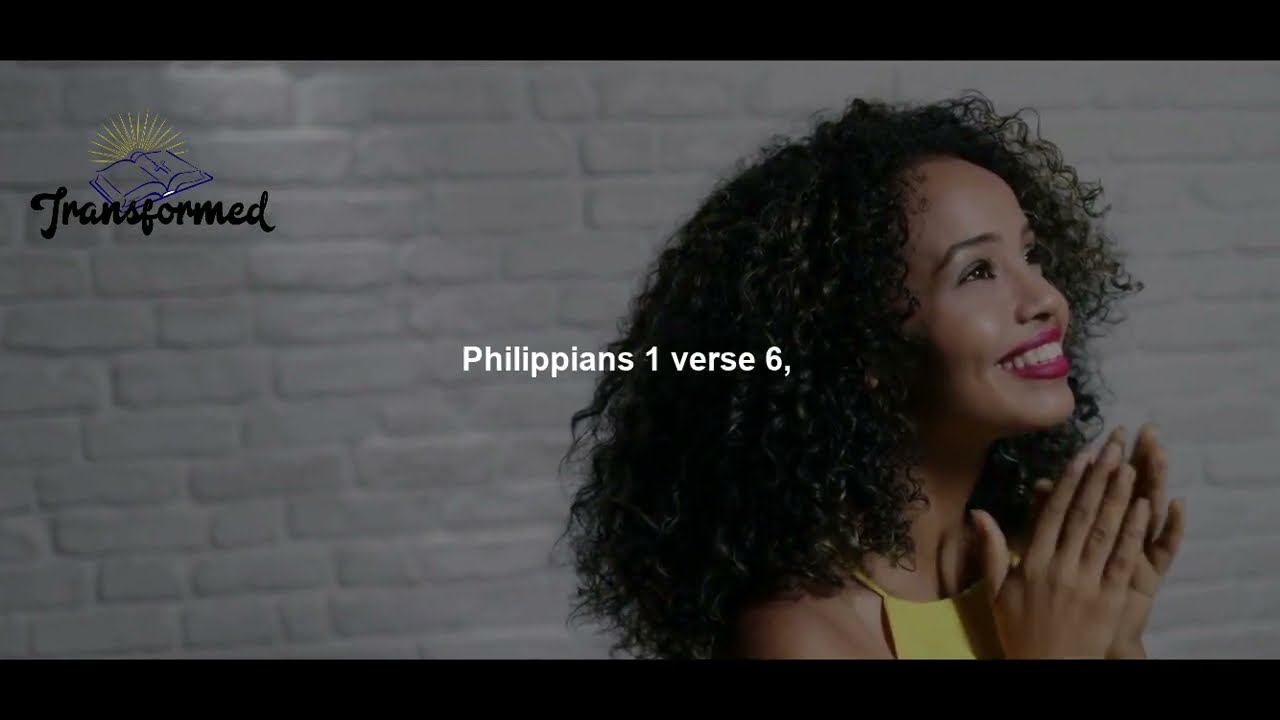In a horizontal rectangular image framed by long, narrow black bars at the top and bottom, a dark-skinned woman with long, puffy black curls and pink lipstick is seen smiling brightly, her teeth visible. She wears a yellow tank top with spaghetti straps and has her hands clasped together near her chin, possibly in a gesture akin to prayer. She looks upward toward the sky, appearing happy and excited. The background features a slightly blurred gray brick wall. In the upper left-hand corner, a logo displays an open book with light shining from behind, accompanied by the word "Transformed" in black cursive writing. In white font, the text "Philippians 1:6," is prominently placed in the foreground.